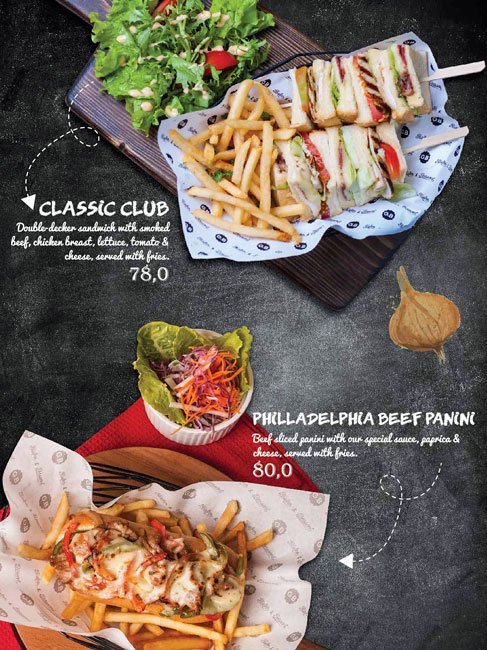In this advertisement for a couple of different sandwiches, the image is divided into two main sections on a black table setup. At the top half, there's a wooden cutting board with a small pot of green salad on the upper left portion, and to the lower right of the board, a wrapper holding a bunch of fries and two sandwiches impaled with spears. A white dotted line spirals out from the left-hand side of the board with an arrow pointing to text that reads "Classic Club Double Decker Sandwich with Smoked Beef, Chicken Breast, Lettuce, Tomato, Cheese, served with fries," priced at 78.0. Just below the right-hand corner of the wooden board is a clip art image of an onion. 

In the bottom half of the image, there's a red napkin with a brown plate sitting on it in the lower left corner. The plate holds a small white bowl containing a salad, in front of which is a basket filled with fries and a visibly cheesy sandwich. An arrow points to text that reads "Philadelphia Beef Panini, Beef Sliced Panini with Special Sauce, Garlic, and Paprika, served with fries," priced at 80.0. The contrasting colors include white, black, tan, brown, red, and green, adding a vibrant depth to this detailed restaurant menu display.